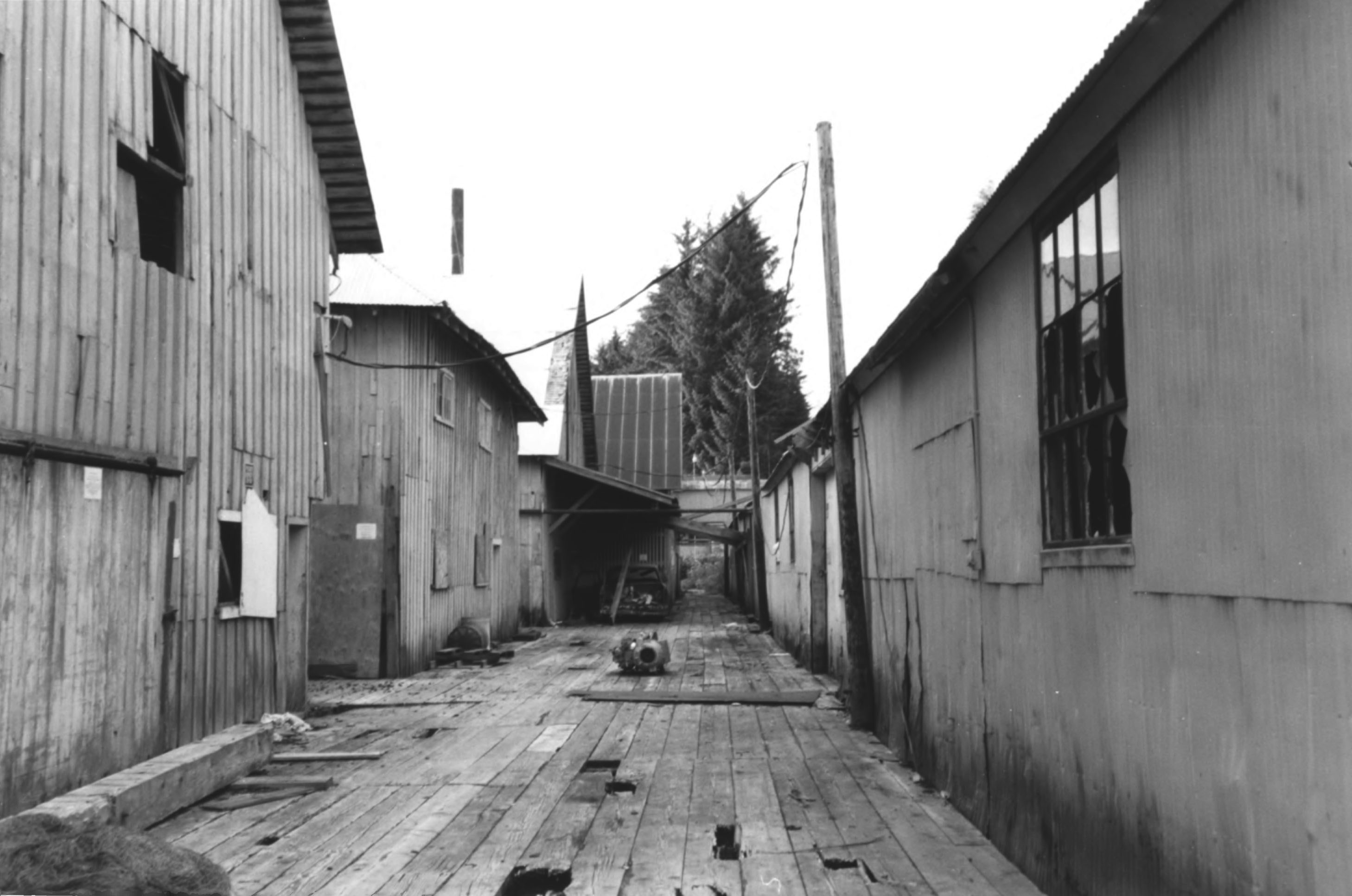The black-and-white photograph, taken in landscape orientation, captures a slightly out-of-focus, deteriorating scene of what appears to be a jetty-like wooden walkway flanked by buildings in severe disrepair. On the right, one-story buildings made of scrap sheet metal feature iron-framed windows, some with shattered glass panes. To the left, a mix of double-story and one-and-a-half-story buildings, resembling barns with sliding doors and corrugated-style pitched roofs, exhibit missing window glass and fading facades. 

Central to the image, a wooden power pole, along with two more further in the background, stretches wires across the walkway to the buildings on both sides. The planked walkway itself is a patchwork of missing chunks and random items, including what appears to be an old, brass scuba helmet lying on its side. Farther along the wooden path, amidst broken planks and errant debris, towering conifer trees loom above a wall that runs horizontally, delineating the background.